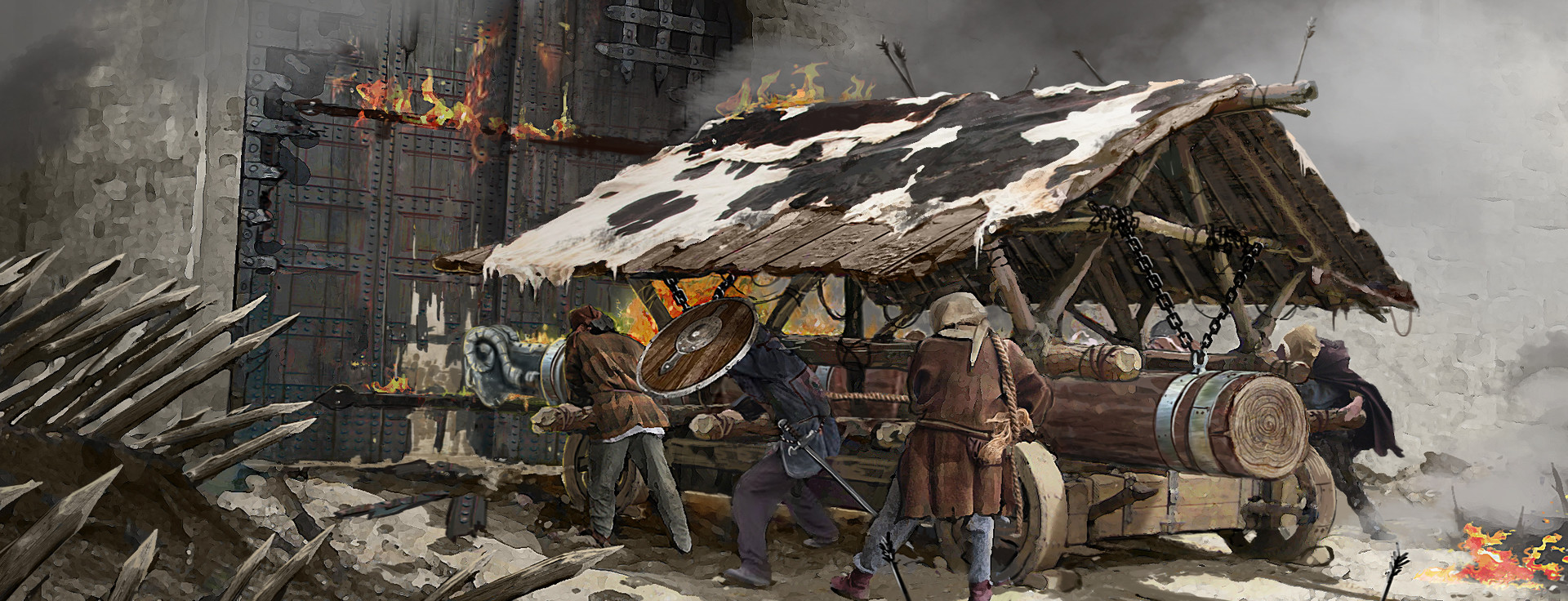The image presents a highly detailed, AI-generated depiction resembling a historic scene with sharp lines and high contrast. It features a group of six men, organized with three on each side of a large, wooden battering ram. The device, designed to break down gates, has a gray head shaped like a bighorn sheep's head, connected to a tree-trunk-like body, and is mounted on wheels. The battering ram is covered by a vaulted, triangular roof made of cow skin for protection. The men, dressed in long coats or brown furs and wielding swords and shields, are attempting to push the ram towards a large iron door of a fortress. Surrounding the scene, there is evidence of a fire starting, both from the front of the vehicle and emerging from the fortress doors, which are engulfed in smoke. Additionally, there are spiky metal elements visible on the left side of the image. The overall aesthetic combines a painted style with a realistic, almost computer-animated clarity, reinforcing the historic, action-packed atmosphere of the scene.